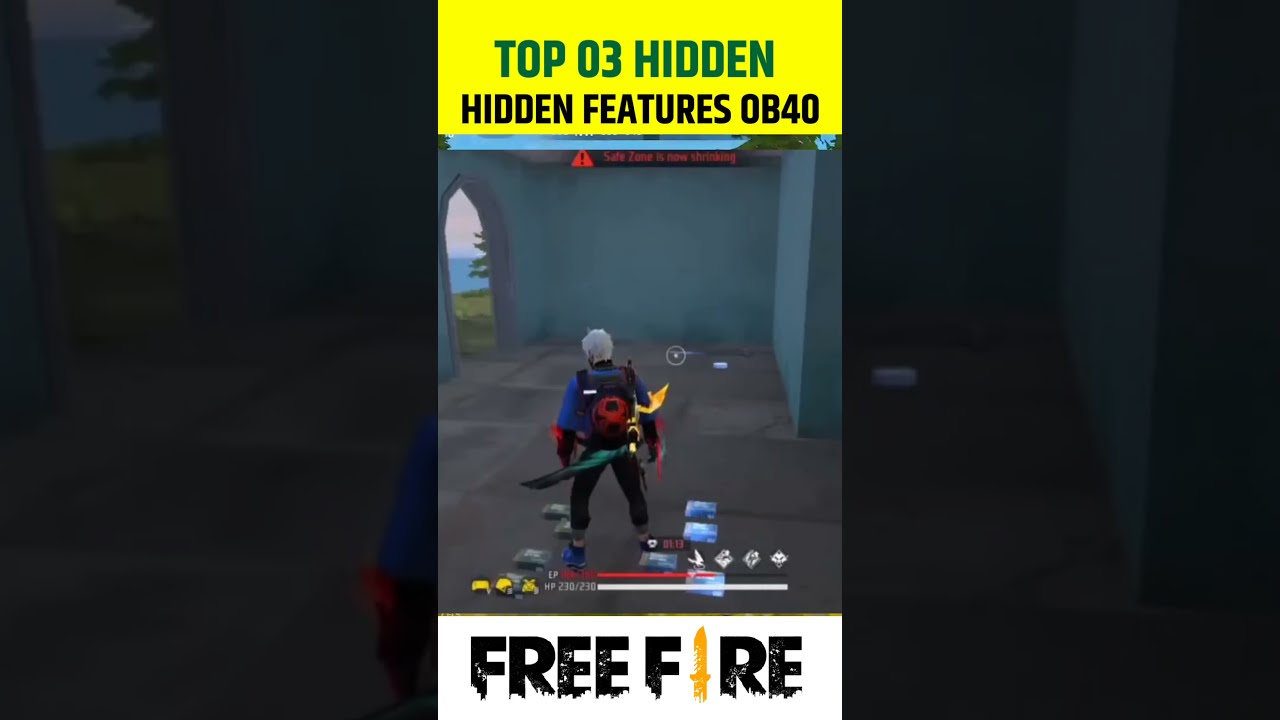This is a screenshot of a video game that could serve as a YouTube video thumbnail. At the top, a yellow banner features the text "Top 3 Hidden" in green print. Below it, "Hidden Features OB40" is written in black. The central image showcases a man in blue long sleeves and a backpack with red accents, facing away from the viewer. He has a sword strapped around his waist extending to the left, wears black pants and blue tennis shoes, and appears to be standing in a courtyard. To his left is a wall with an arched entryway, revealing grass and an ocean beyond. The character has gray hair and possibly carries a green and yellow weapon on his back. Below him are a life bar (red) and an HP bar (white) indicating "230 out of 230," along with some unreadable icons. At the very bottom, the text "Free Fire" is displayed in yellow, where the 'I' is stylized as a knife. The sides of the image are black and slightly opaque, possibly showing faint hints of trees or other surroundings.